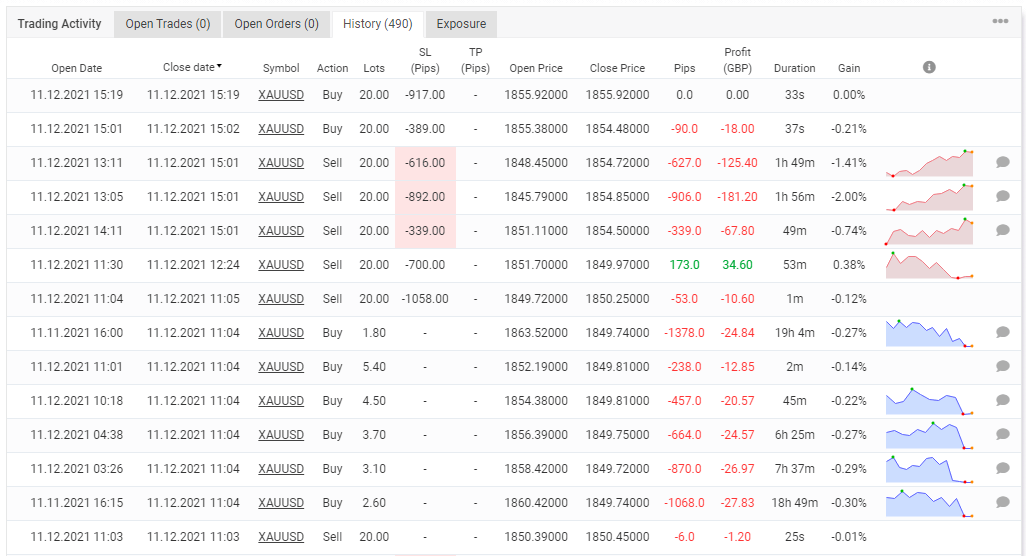The image depicted is likely a screenshot from a stock trading or forex trading platform. This detailed image predominantly features a monochromatic scheme of white and gray, interspersed with red and green numerical data. The top section of the image shows a navigation menu with the tabs: "Trading Activity," "Open Trades," "Open Orders," "History," and "Exposure." The selected tab "History" is accompanied by a parenthetical figure indicating "(490)."

Below the navigation, the display lists several trades with their respective details such as open and closed dates, trading symbol, action performed (buy or sell), and the number of lots traded. The open dates span the 11th and 12th of November 2021, while the closed dates are unified on November 12th, 2021. Each trade involves the symbol XAUUSD. The listing details include:

- Open Dates: November 11th and 12th, 2021 
- Closed Date: November 12th, 2021 
- Symbol: XAUUSD
- Actions: Bought/Sold
- Lot Sizes: 1.80, 5.40, 4.50, 3.70, 3.10, 2.60, and 20

Additional columns detail the terms TP (Take Profit) and PIPs, however, specific figures for TP are not displayed. The opening and closing prices for the trades are noted along with the calculated PIPs. The resulting profit or loss is visually represented by negative (red) or positive (green) numbers, with only one instance of a positive green number in this dataset.

Moreover, the "Duration" column displays a variety of figures, likely indicating time intervals of trades, followed by the "Gain" column, which is illustrated with either red or blue graphics. Some entries also feature a gray chat bubble icon, possibly indicating accompanying notes or comments about the trades.

Overall, the image offers a comprehensive overview of trading history with detailed transactional data relevant to the symbol XAUUSD.